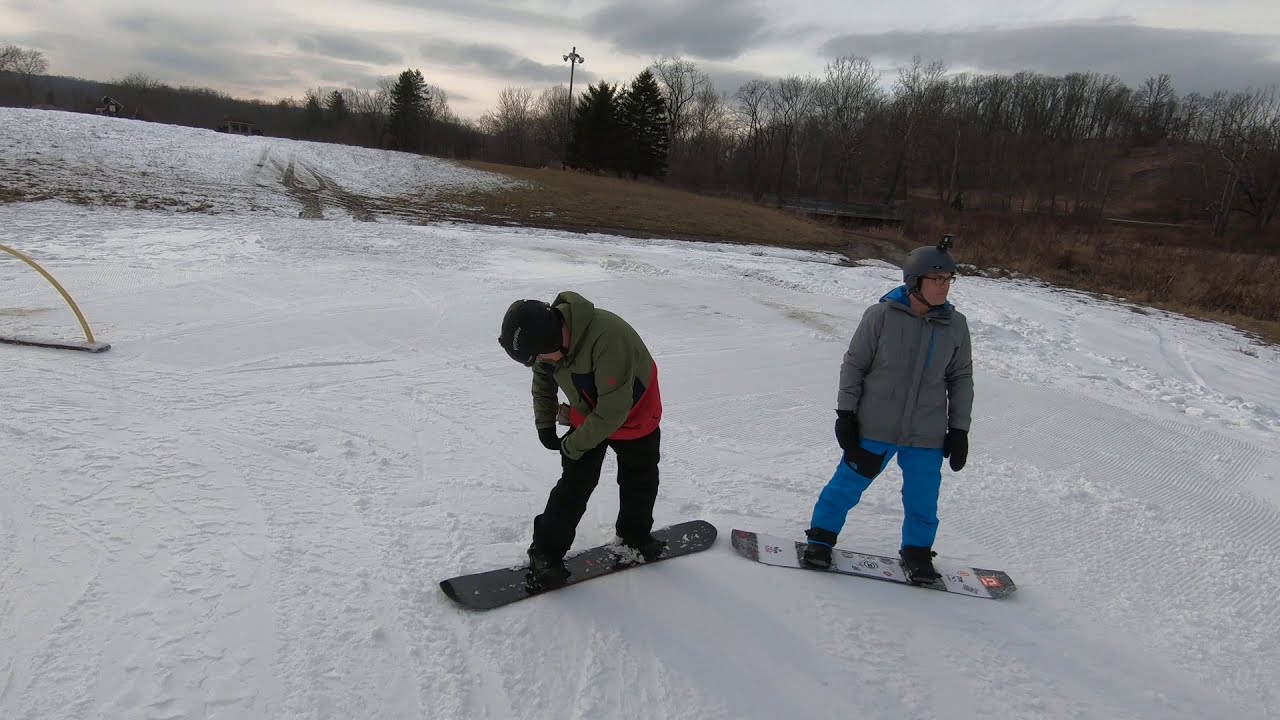The photograph captures a slightly elevated snow-covered slope marked by various tire tracks and skid marks, indicating it's an active area. The sky is a light gray adorned with darker gray clouds. In the distance, a tree line comprises mostly leafless trees, typical of winter, with some evergreen pines still showing their green needles. Scattered patches of dark brown grass are visible where the snow has melted. In the foreground, two individuals stand on snowboards. The person on the left sports a black snowboard, black boots, black pants, a green and red jacket, and a black helmet, appearing to look down toward a pocket on their pants. To their right, the other person stands on a white and black snowboard, wearing black boots, blue pants, a gray jacket, and a gray helmet with a black camera mounted—possibly a GoPro. Both appear poised to descend the slope.